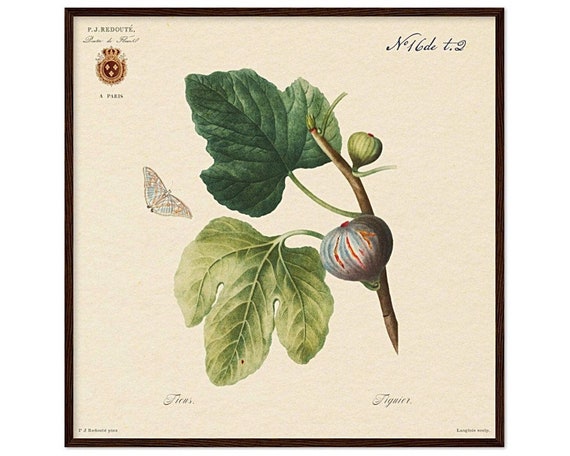This image is a detailed botanical illustration, possibly from a historical scientific journal or field guide. At the center of the image is a short plant with a dark green, tri-sectioned leaf at the top and a lighter, paler leaf below. The plant has a slender black stem. Along the stem, there are two distinctive bulbous flowers: a small pale green bud near the top and a larger, mature bulb with striking blue and red stripes below it. The plant is set against a beige background, which some may perceive as white. A small butterfly accompanies the plant, adding a touch of delicacy to the composition. Additionally, there is some text, which appears to be the plant's name and other information, though it's difficult to read. A royal emblem is positioned in the upper left corner, and there's a notation, possibly "number one," in the upper right, suggesting that this is a carefully documented and classified image from a significant source.